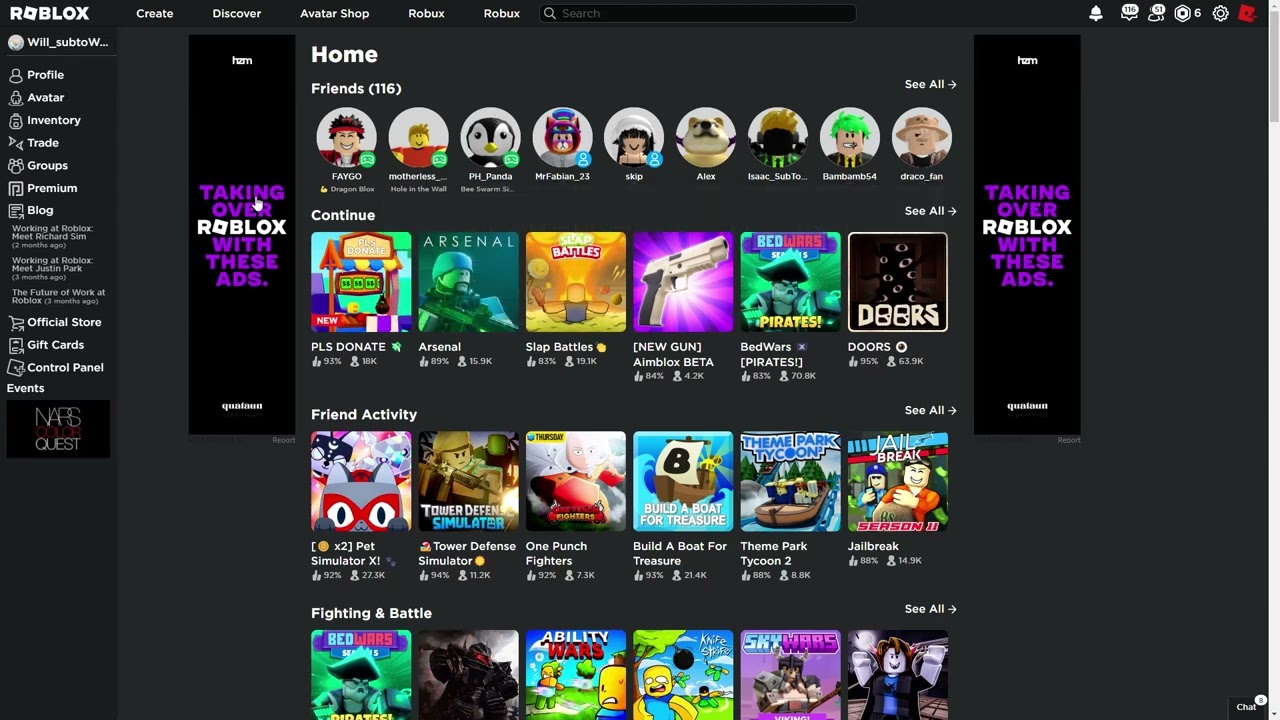This image captures the home interface of Roblox, set against a dark gray background. In the top-left corner, the Roblox logo is prominently displayed. Just below, the username appears as "will_sub_to_D...". The vertical menu on the left lists several options: Profile, Avatar, Inventory, Trade, Groups, Premium, Blog, Official Store, Gift Cards, Control Panel, and Events.

The main interface is divided into rows. The top row showcases "Friends (116)" with their profile pictures and usernames arranged neatly. Directly below, the "Continue" section highlights recently played games, which include: Please Donate, Arsenal, Slap Battles, New Gun, Blox Beta, Bed Wars, Pirates, and Doors.

Further down, "Friend Activity" lists games that friends have been playing, such as Pet Simulator X, Tower Defense Simulator, One Punch Fighters, Build a Boat for Treasure, Theme Park Tycoon 2, and Jailbreak. Below this, the "Fighting and Battle Games" section offers a glimpse of various games, though their names are cut off in this view; the promotional images for each game are visible.

On both the left and right sides of the interface, an advertisement reads, "Taking over Roblox with these ads," featuring a black background and purple text, with "Roblox" highlighted in white.

At the top of the screen, a navigation bar includes options for Create, Discover, Avatar Shop, Robux, and a search bar, alongside several other user interface icons.